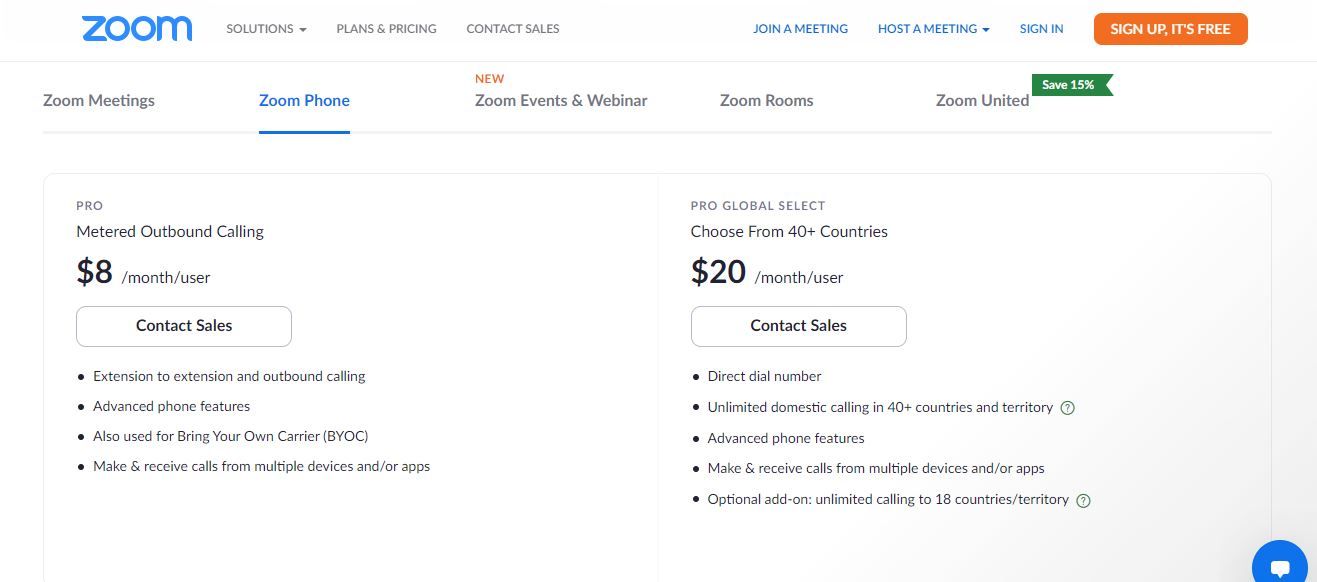This detailed caption describes a horizontal, rectangular screenshot of a Zoom webpage. In the top left corner, the word "Zoom" appears in blue, followed by a menu with a drop-down option labeled "Solutions." Next to it, in black text, are "Plans & Pricing" and "Contact Sales." On the right side of this section, blue text reads "Join a Meeting" and "Host a Meeting" with a drop-down or button labeled "Sign In." Further right, there's an orange button with white text that says "Sign Up, It's Free."

Below this, a secondary menu begins with "Zoom Meetings" and "Zoom Phone," the latter highlighted in blue to indicate selection. The next section shows the word "New" in orange above "Zoom Events & Webinar." This is followed by sections for "Zoom Rooms" and "Zoom United," the latter featuring a green symbol that says "Save 15%."

The content then focuses on two Zoom Phone options. The first option, "Pro," offers metered outbound calling at $8 per month per user, accompanied by a "Contact Sales" button. Four bullet points list features: Extension to Extension and Outbound Calling, Advanced Phone Features, Compatibility with Bring Your Own Carrier (BYOC), and the ability to make and receive calls from multiple devices or apps.

To the right, the "Pro Global Select" option is detailed: at $20 per month per user, it offers choosing from 40+ countries. This plan includes a "Contact Sales" button and five bullet points, listing: Direct Dial Number, Unlimited Domestic Calling in 40 Countries and Territories, Advanced Phone Features, the ability to make and receive calls from multiple devices or apps, and Optional Outbound Unlimited Calling to 18 Countries/Territories. 

Finally, in the bottom right-hand corner, there's a blue messaging icon.